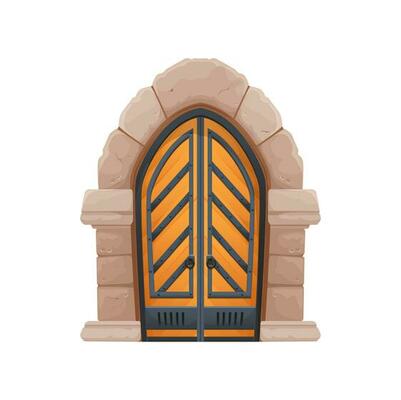The image showcases a cartoon-style archway constructed from illustrated stone blocks. At the base of the arch, there are three levels of light tan, taupe-colored stones that are accented with some pale pink and darker pink tones. The base is depicted with three cylinders resembling round, cinder block stones. The arch itself is formed from larger, round stones that alternate between pale pink and light pink hues. In the center of the archway is a double door, distinguished by its orange color and framed with a greenish-black outline. Each door is detailed with intricate diagonal lines that draw towards the black doorknobs located at the center junction. At the bottom portion of the doors, a blue-gray stripe functions almost like a kick plate, while similar blue stripes run down the center and around the top of the panel, following the shape of the door in an up-and-down zigzag pattern. The overall background of the image is a clean white, emphasizing the vivid, playful style of the archway and door combination, hinting at a construction that could be made from plastic or clay to resemble a child’s play structure.